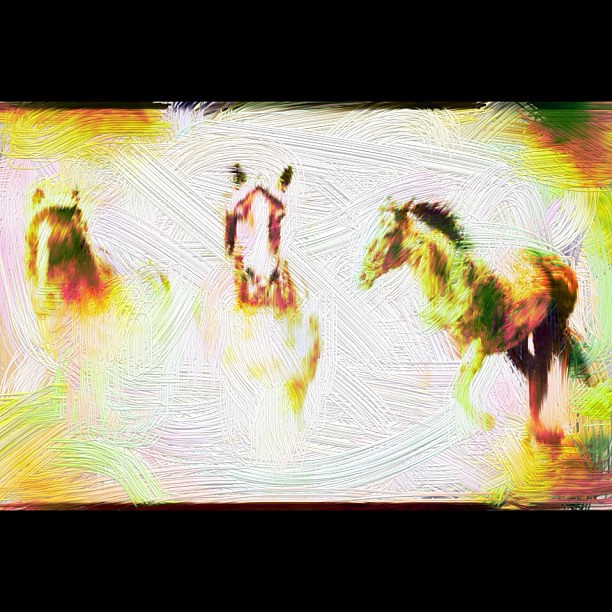This is an abstract watercolor painting depicting three horses amidst a vibrant, textured background. The artwork primarily features vigorous, deep paint strokes that move in various directions, creating a sense of dynamic motion and energy. The painting is largely white with splashes of blue, green, yellow, and red towards the edges, contributing to its colorful ambiance.

In the center, three horses are portrayed with varying degrees of detail. The left and center horses face forward, their forms rendered with loose, indistinct outlines that blur into the background. The horse on the right is more detailed, facing to the left, and appears to be in mid-run. This horse's body, especially its legs, blends seamlessly into the textured backdrop, accentuating the fluidity and wildness of the scene.

The overall composition is framed by broad black banners at the top and bottom, grounding the otherwise ethereal and spirited depiction. The horses themselves are painted in shades of brown, red, green, and yellow, with the two facing the viewer adorned with distinctive white blazes. The entire piece exudes a sense of motion and freedom, capturing the essence of wild horses in their natural, untamed state.